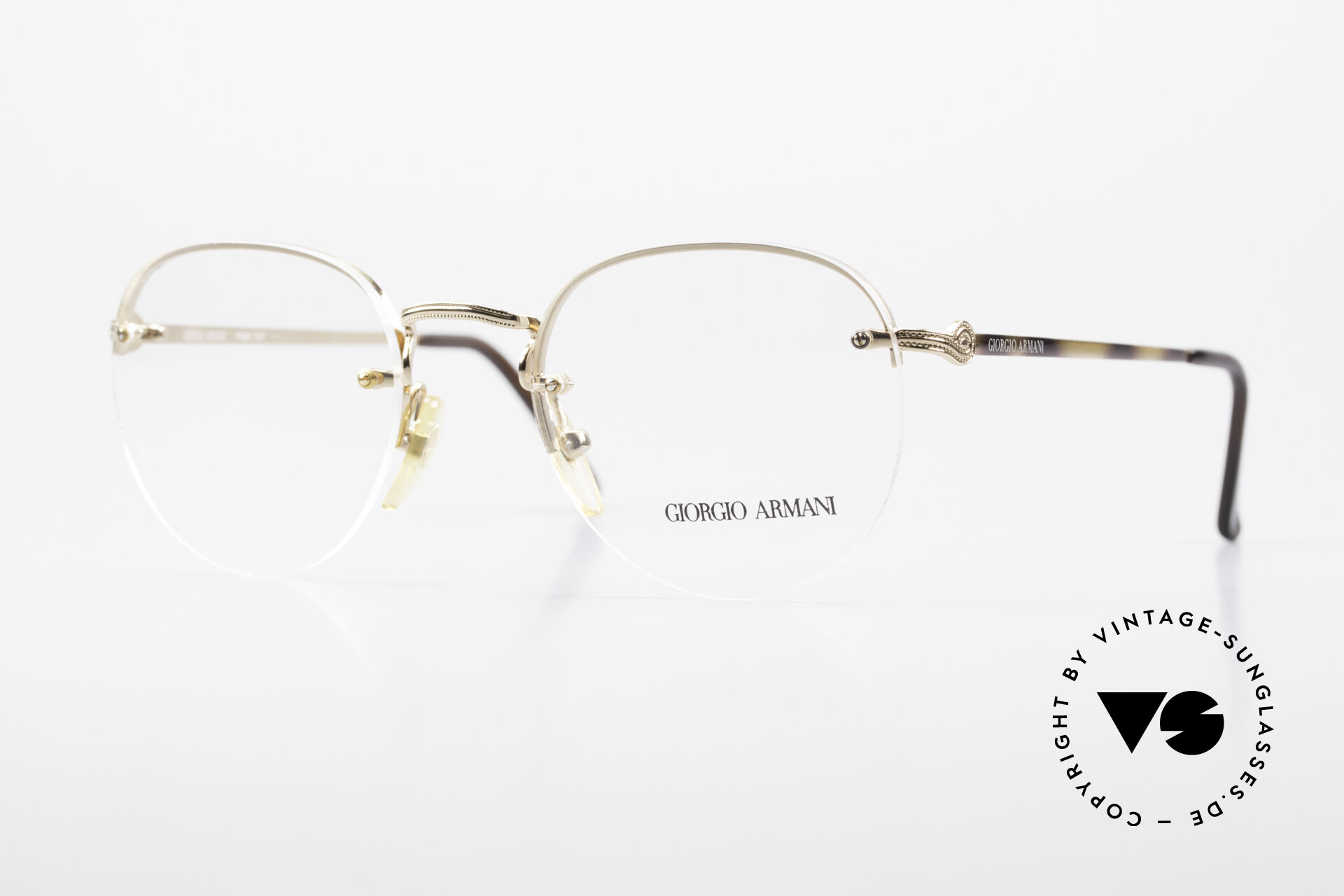This is a detailed, up-close photo of a pair of Giorgio Armani glasses, prominently displayed against a white background. The glasses, which have thin, barely visible frames, appear to be predominantly clear with a tortoise shell pattern of tan and light brown hues. They feature round lenses with the Giorgio Armani branding visible on the front of the right lens. The thin ear pieces are accented with chrome or silver decorative parts, including the nose piece. In the bottom right corner of the image, there is a circular advertisement watermark that reads "copyright by vintage-sunglasses.de" and features the VS emblem, which includes a logo resembling an upside-down triangle within a circle. The focus on the glasses and the high contrast of the white background suggest that this image is likely intended for an advertisement.